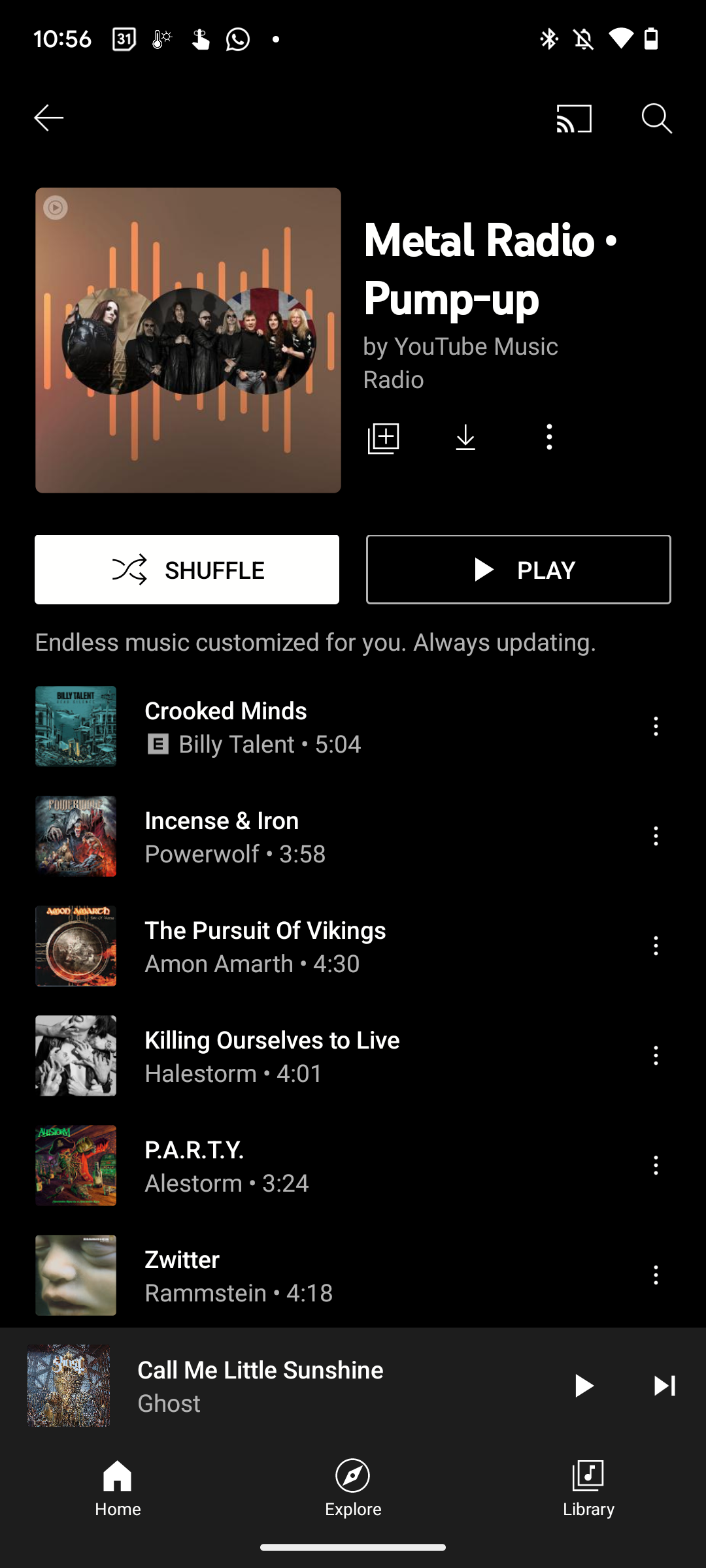The image displays a smartphone screen, featuring various icons and information against a black background with white or gray text. At the top left, the time is shown as 10:56, along with a temperature icon indicating 31°. Next to it, there's a reminder icon. Towards the top right, there are icons for a missed call, Bluetooth connectivity, and a notification bell with a diagonal line through it, indicating no notifications. The Wi-Fi icon is present, along with a battery indicator showing 50% charge.

Below this section, on the left side of the screen, there's a left-facing arrow. On the right, there is a square with lines in its bottom left corner, the function of which is unclear. Adjacent to it, there is a search icon depicted as a magnifying glass.

Following this, there is an image of what appears to be a band. To the right of this image, text reads "Metal Radio, Pump it up" by YouTube Music Radio. Additionally, there are icons for adding the station to favorites (a plus sign in a square), downloading (an arrow pointing down to a line), and more options (three vertical dots).

Further down, there are two prominent buttons: a white "Shuffle" button with a black icon and text, and a black "Play" button with a white play arrow icon and outline.

A description below these buttons reads, "Endless music customized for you, always updating."

The screen then lists a series of songs with accompanying images and text in white and gray fonts, featuring tracks like "Crooked Minds" by Billy Talent, "504," and "Incense and Iron" by Powerwolf.